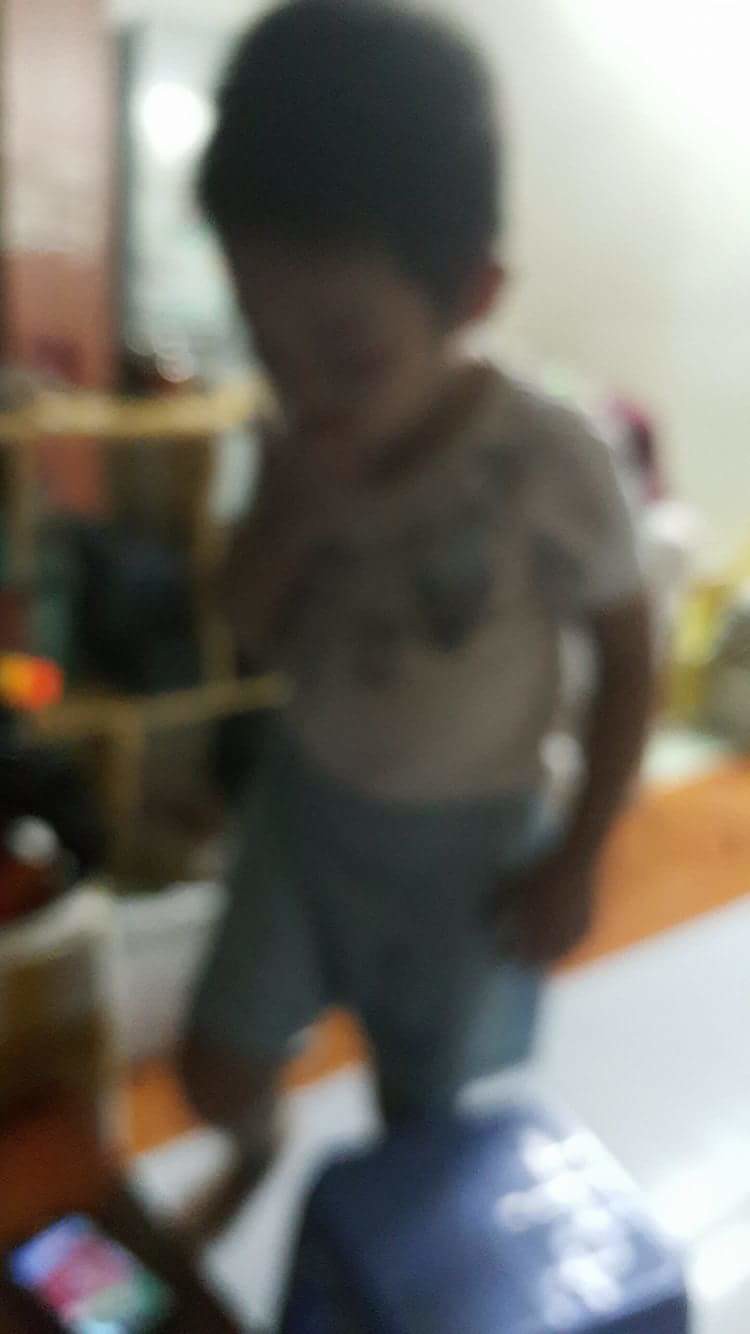The image shows a young child, estimated to be between 4 and 10 years old, standing in front of the camera and facing slightly to the left. The child, who has dark hair, is raising its right arm towards its mouth while looking down, giving the impression of either a contemplative or distracted moment. The child is wearing a brown shirt with indistinct patterns and blue pants that seem to have a greenish hue on one side. The background reveals a mixture of objects and colors: a wooden shelf with various items, including blue, green, orange, white, and red colors, and a wall that transitions from green to white towards the upper right-hand side. In the foreground, on the floor in front of the child, is a small screen that appears to display an image or a game, though it is difficult to make out due to the blur. Additionally, there are indistinct objects like a blue box and what might be a box of tissues in the lower left corner. The entire image is very blurry and out of focus, further obscuring the details of the scene.